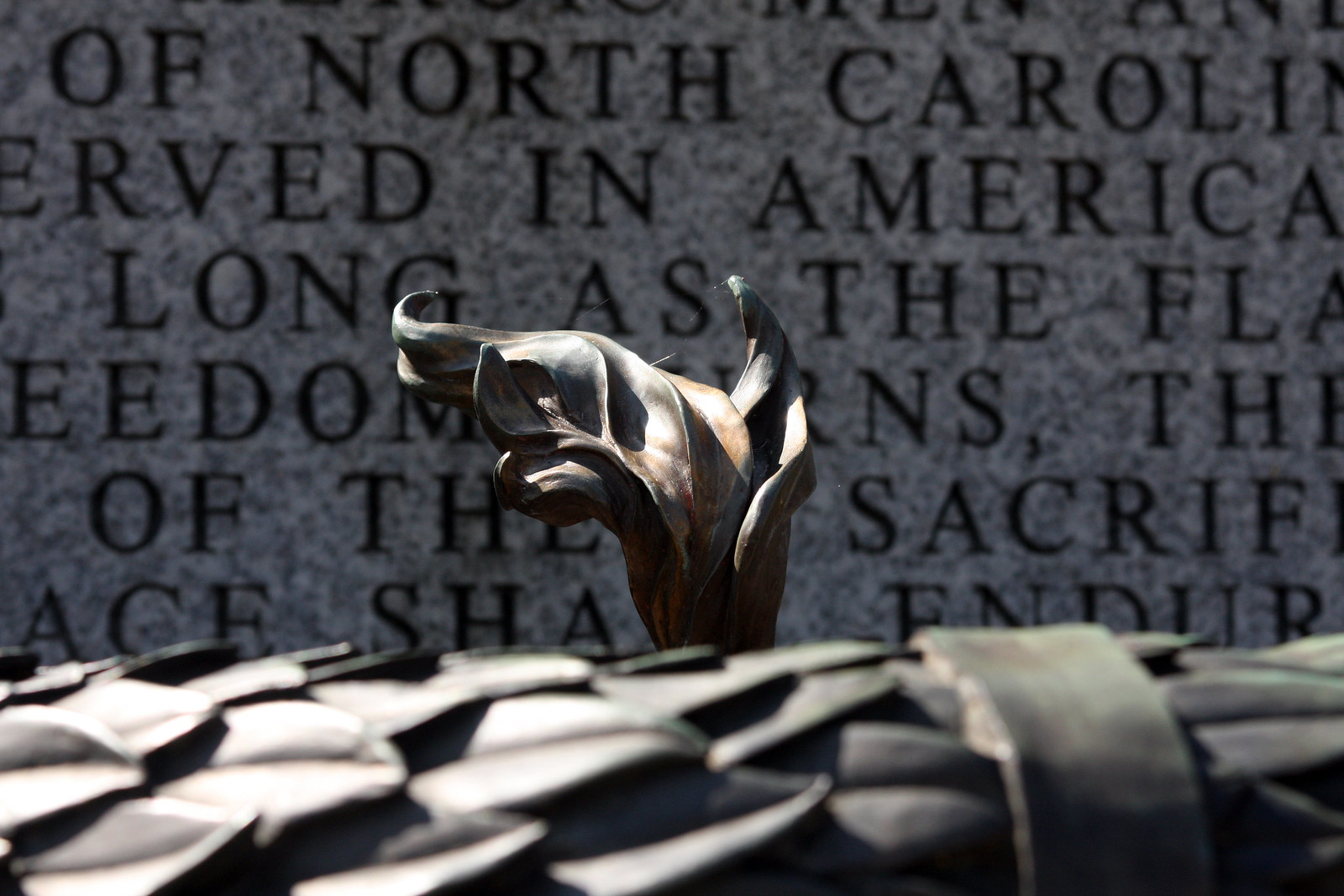The close-up image captures a detailed section of a bronze-colored metal sculpture, most likely part of a larger memorial dedicated to fallen soldiers. The sculpture, a flame-like structure appearing to rise from a spiny base, displays intricate grooves and a small spider web delicately woven between its edges, emphasizing the high-quality focus of the photograph. Behind the sculpture, a granite wall serves as the backdrop, partially revealing bold, black inscriptions such as "North Carolinian," "served in America," "freedom," and "sacrifice." These elements suggest that the setting is an outdoor military memorial in North Carolina, with the sunlight casting reflections on both the flame and the surface it rises from, adding to the solemn reverence of the scene.